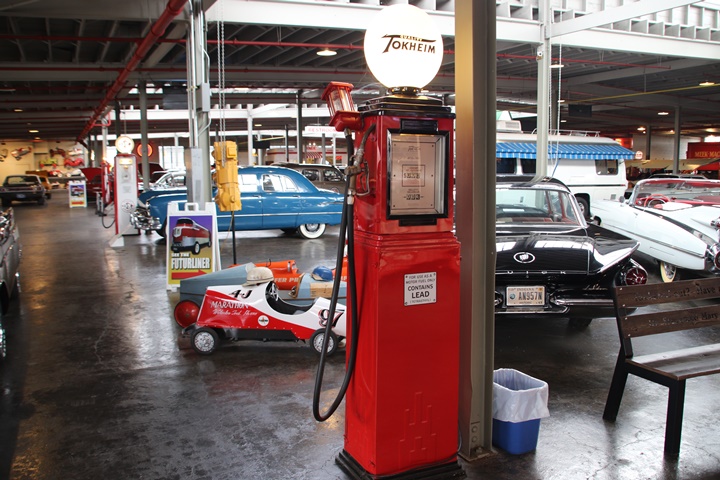Inside a large, polished cement floored warehouse, this detailed photo depicts a vintage car museum. The central focal point is a bright red, old-fashioned gas pump from the 1940s or 50s, identified by the illuminated white glass bowl on top that says "Tokheim." Surrounding the pump, there are meticulously maintained, shiny cars from the 50s and 60s, including a distinctive blue four-door car with white wall tires and a white convertible. Among them, a notable Volkswagen van has been converted into a recreational vehicle, featuring a blue and white awning. Also present are toy pedal cars for children from the era, including a red and white mini race car adorned with "4J" and "87." Additional elements such as a wastebasket and a bench sit beside the gas pump, enhancing the nostalgic and historical ambience of the scene.